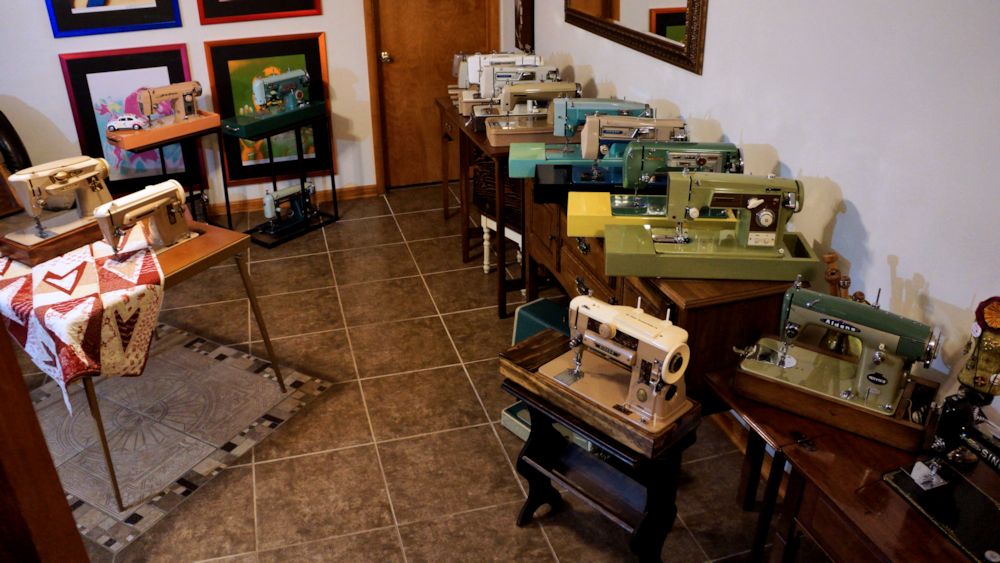This photograph depicts a vintage sewing room filled with a diverse collection of old sewing machines. There are approximately twelve sewing machines of various shapes and colors, including white, gray, brown, green, and turquoise. The machines rest on an eclectic mix of furniture, including wooden desks, dressers with drawers, and small tables. One orange table stands out among them. The room features brown tile flooring and white walls adorned with colorful frames that contain art, although the details of the artwork are not visible. A wooden door is present in the back wall. On the left side of the room, there are three long desks, each hosting multiple sewing machines. Among the sewing paraphernalia, there's a white model car and a quilted blanket with heart designs. The entire setup evokes a nostalgic atmosphere, suggesting these sewing machines are vintage models.